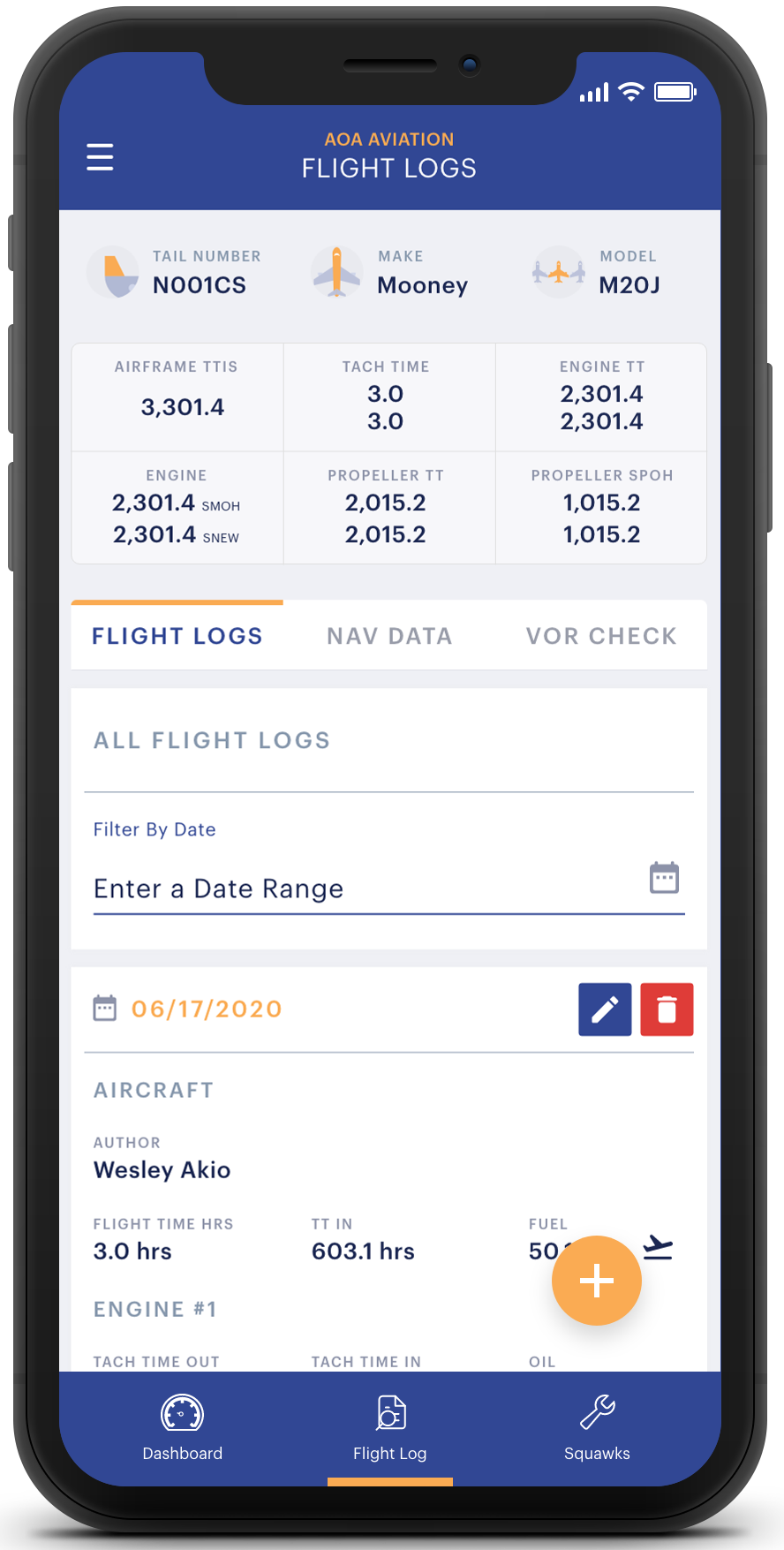The image shows a mobile phone screen displaying a website related to aviation. The phone's battery is fully charged at 100%, as indicated by the white battery bar at the top of the screen. The connection status is excellent, displayed by three horizontal bars on the left.

The website header reads "AOA Aviation" in orange text. Below this, the menu options include "Flight Logs" highlighted in blue, "Nav Data" in gray, and "VOR Check" in gray. The background of the website is light gray.

The main content begins with sections labeled "Tail Number," "Make," "Model," "Airframe," "Tack Time," "Engine," "Engine-Propeller," and "Propeller." A gold bar at the top of the "Flight Logs" section highlights various flight logging features.

Beneath this bar, the subheading "All Flight Logs" appears, along with an option to filter logs by date. There is a text box on the right where a date range can be entered. Details of a specific flight from 06-17-2020 are listed below, including aircraft information and navigation boxes: a blue box with a crayon icon for editing and a red box with a trash can icon for deletion. The author of the log is Wesley Akio, with recorded flight time of three hours, TTIN (Total Time in Service) of 603.1 hours, and partially visible fuel information showing "50."

Moreover, there is an orange circle with a plus sign, next to which is an airplane icon, indicating an option to add new entries. At the bottom, a blue navigation bar shows "Dashboard," "Flight Log," and "Squawks," with "Flight Log" underlined in orange.